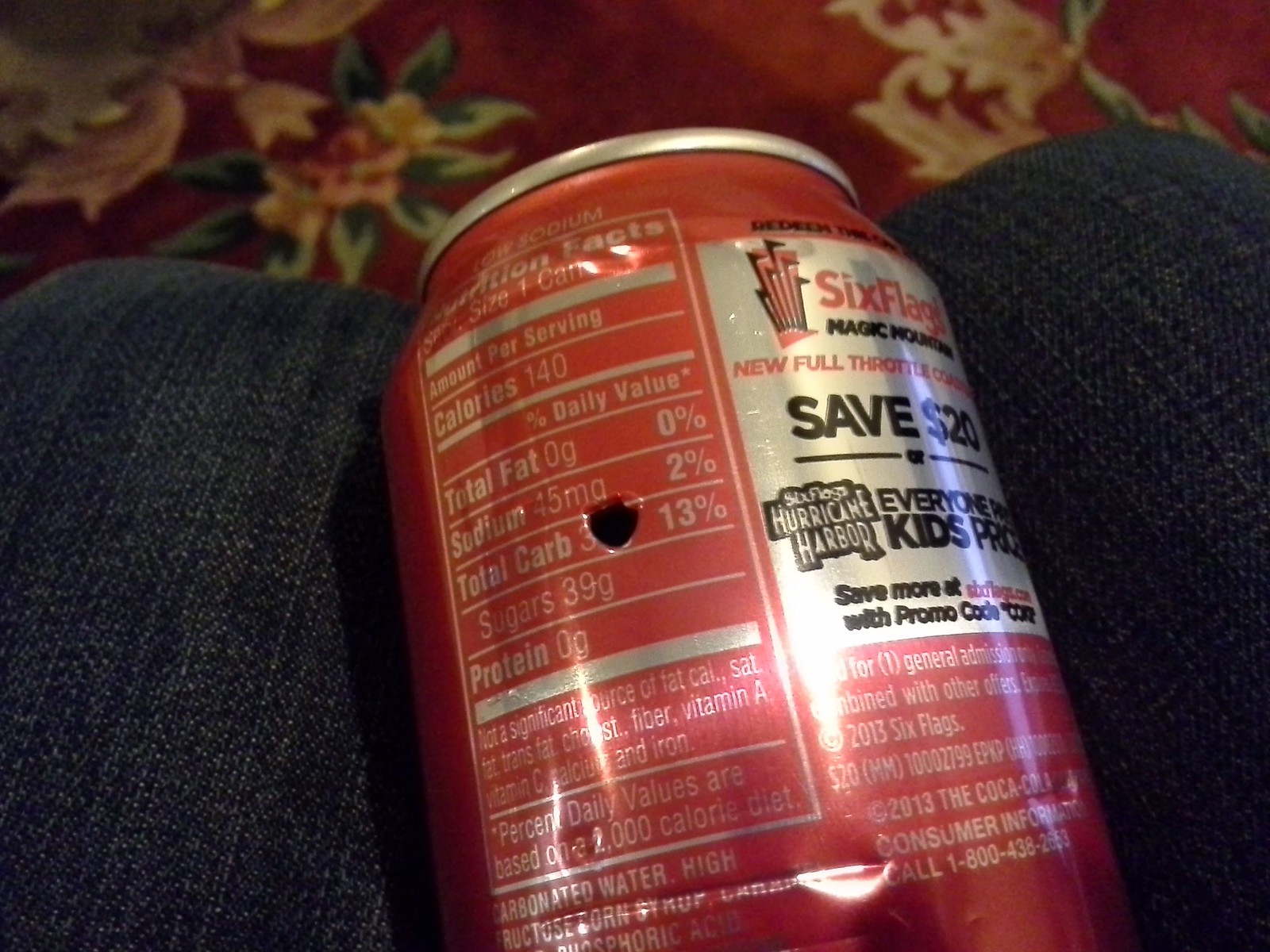The image depicts a red soda can, typical of popular cola brands, prominently featuring a silver advertisement box with red letters promoting "Six Flags" and black letters partially revealing the words "Magic Wonderland." The message appears to be part of a promotion offering a $20 savings for Six Flags Hurricane Harbor. The can has suffered a puncture wound, likely made by a pen or a similar pointed object, which has created a hole through the detailed nutritional facts on the side of the can. The can's silver rim is clearly visible, and it is resting on the lap of an individual wearing dark blue jeans, positioned just above their knees. The surrounding setting includes a glimpse of the carpet underneath the legs, characterized by a red base with intricate green, pink, and light-colored floral patterns.